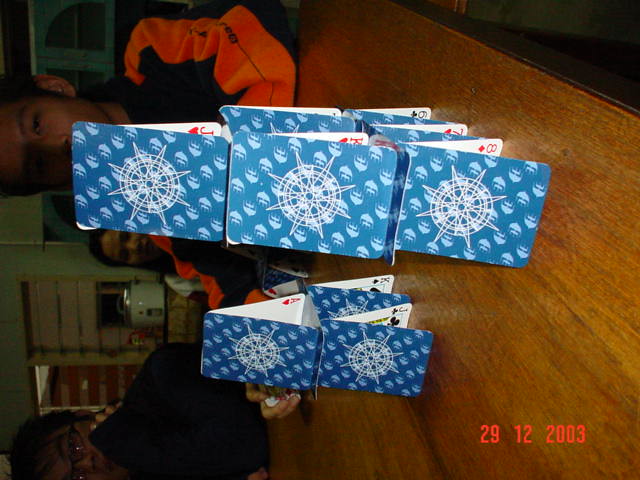The image is oriented sideways, featuring a brown table with an intricate structure built from playing cards atop it. In the foreground, the cards display blue backs adorned with white stars and small fish motifs. At the base of the main card structure lies a broad foundation of cards, topped by two subsequent layers: the second one prominently featuring a King, and the pinnacle adorned with a Jack. Visible numbers on the cards include 8, 7, and 6.

To the left of the main card structure stands another, smaller construction, consisting of a foundation of three cards and an upper layer of two cards. Within this secondary arrangement, an Ace, a King, and a Jack are discernible.

Three individuals are seated in the background, possibly in a kitchen distinguished by green walls and striped patterns along the back. The boy on the left wears a blue sweatshirt, while the other two people don red sweatshirts. Additional details include a pot or kettle on a countertop and paintings hanging on the right wall. An open door is visible at the rear of the room. Notably, the bottom of the photograph is marked with the date "29-12-2003." The right side of the brown table is highlighted in black.